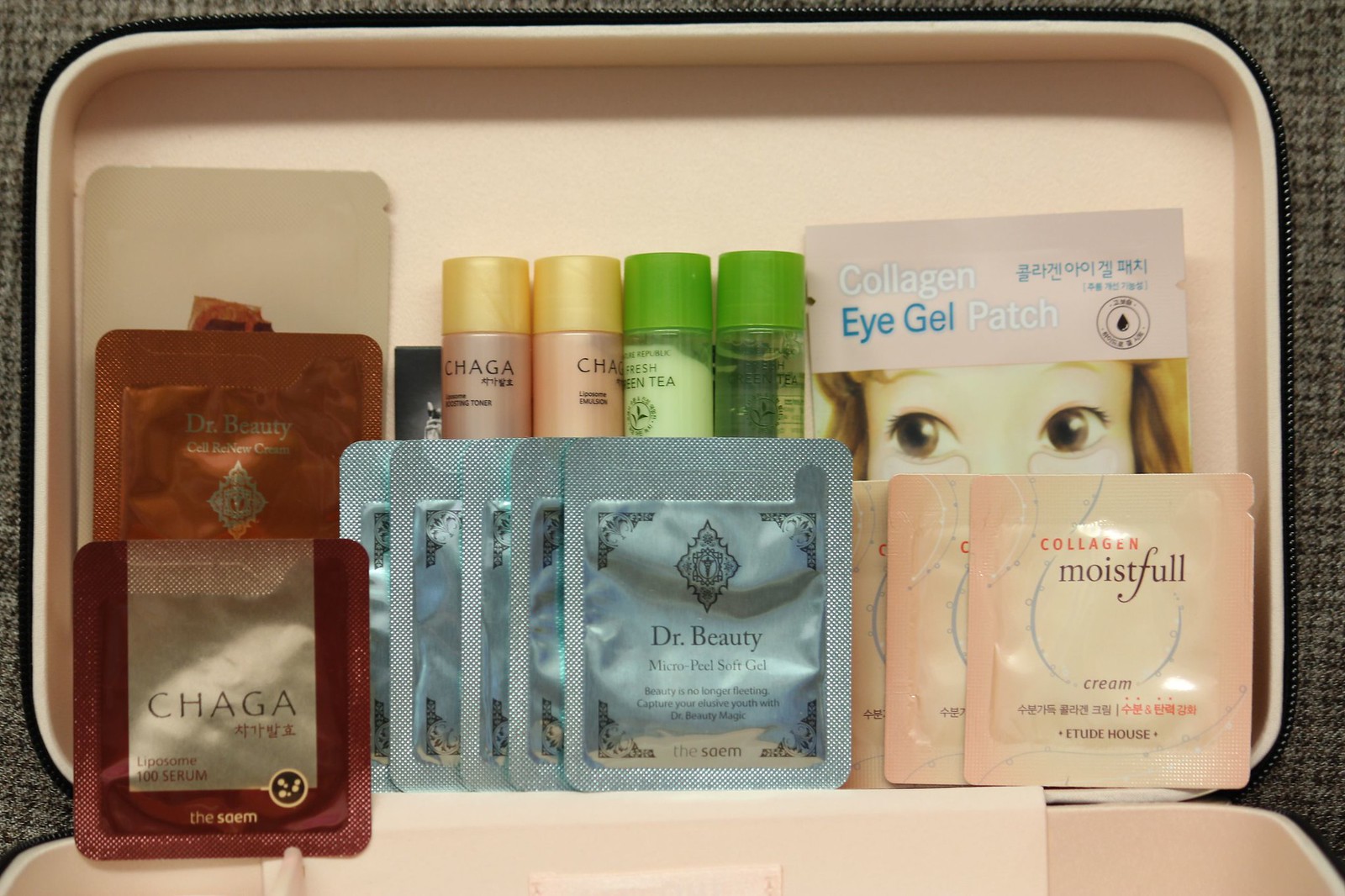A fabric-covered surface, possibly a couch or a chair, serves as the backdrop for a meticulously organized collection of face products contained within a sleek, light pink case with a black rim, designed to be zipped up. The interior of the case showcases a variety of skincare items primarily consisting of patches and foil packs. Notably, the upper left corner features a Dr. Beauty Cell Renew product in distinctive red plastic foil, though the precise item is unidentified. Another red plastic foil pack labeled "Chaga Liposome" accompanies it. There are also four Chaga bottles; the first two exhibit a pinky-tan color with yellow caps, while the next two are green with matching green caps. Additionally, there's a collagen eye gel patch, along with five blue foil packs from Dr. Beauty and four collagen moisturizing cream packs from Etude House, completing the array.